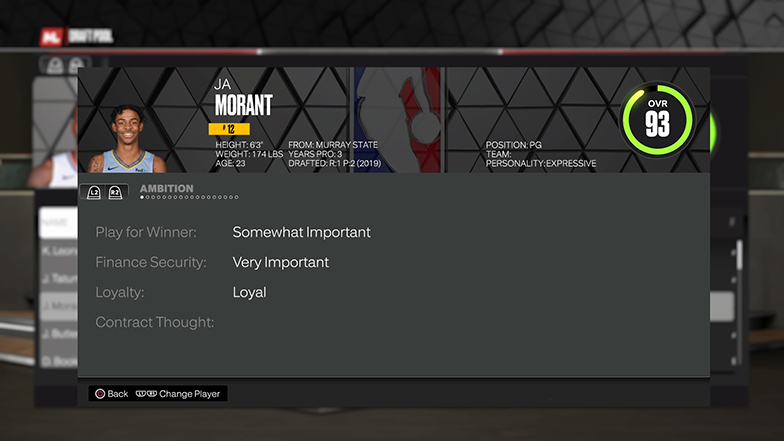This is a detailed screenshot from a sports website, prominently featuring an active pop-up menu that blurs out the dark gray, cross-hatched background of the webpage. The focal point of the screenshot is a light gray pop-up menu. At the top of this menu is a large rectangle with cross-hatching, centered within which is the iconic NBA logo—a white silhouette of a man holding a basketball against a blue and orange backdrop.

In the lower left corner of this rectangle, there is a high-quality photograph of a young African-American man in his early 20s. He is smiling and wearing a blue basketball jersey, and there are visible tattoos on his right arm. He has short black hair. Beside this photograph, white text identifies him as Ja Morant. Below this identification, a yellow rectangle with black text displays his jersey number, "12." Further details about Ja Morant are provided in black text beneath this yellow rectangle, including his height (6'3"), weight (174 pounds), age (23), college (Murray State), professional years (3), and draft year (2019).